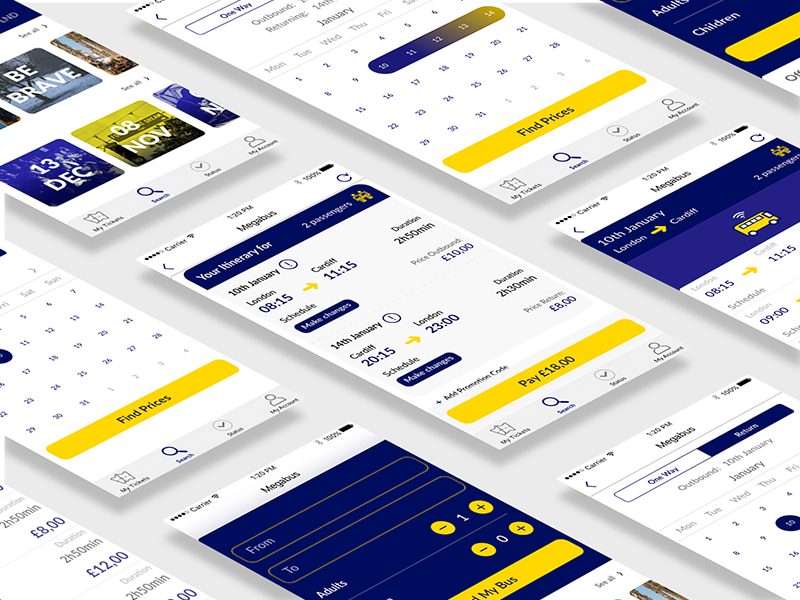This image showcases a promotional page for an app, prominently featuring multiple mobile device screens arranged in rows from an overhead perspective. On the left side, a screen displays a calendar interface, indicating an option to select dates for a trip. The central section features a variety of screens: one shows motivational text, "Be Brave," with dates marked for December 13th and November 8th, while another screen displays an itinerary for two passengers detailing an upcoming trip, with the top bar prominently displaying "Megabus." Below, a secondary Megabus screen can be seen indicating payment processing. On the rightmost top section, another screen shows a yellow bus graphic under the Megabus branding, suggesting trip planning. In the top-center area, a screen presents a calendar with an instruction to "find prices below," emphasizing the app’s price-checking feature.